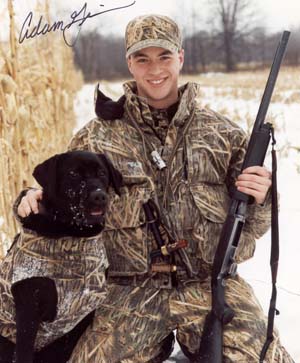The photograph captures a young hunter and his black Labrador posing in an outdoor snowy setting. The hunter, dressed from head to toe in reed-like camouflage with a matching hat, jacket, and pants, smiles warmly at the camera, his curved eyes and visible teeth reflecting his joy. Seated with a large rifle upright on his lap, he's petting his camouflaged-vest-wearing dog, his hand resting gently on the dog's neck. The dog's dark coat contrasts against the snowy ground and barren trees in the background. Additional gear, possibly a flashlight or dog call, is visible around his neck, adding to the detailed preparedness of his hunting attire. The scene is set with dried weeds behind him, emphasizing the wintery outdoor environment.